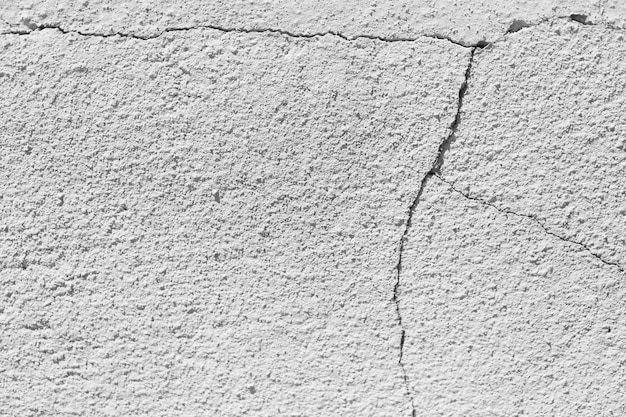This image is a close-up, detailed view of a roughly textured, light gray concrete or stucco wall. Prominent in the image is a network of black jagged cracks. The main crack starts near the top left corner, extending diagonally in a fractured, spiderweb-like pattern towards the top right. About an inch past the center, a vertical crack branches off, curving slightly outward before continuing down to the bottom of the image. From this vertical line, approximately mid-way, a thinner crack angles outward toward the right side. Overall, the image captures intricate and natural crack formations against the rough, coated surface of the concrete.